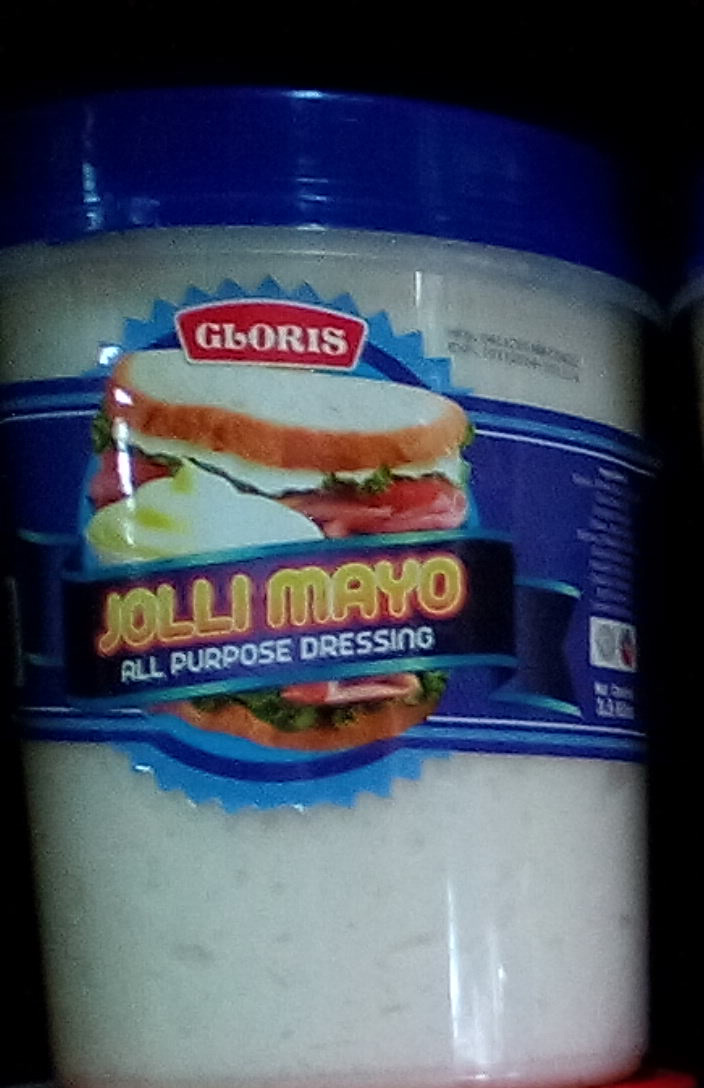This close-up photograph, set against a solid black background, features a clear plastic jar of mayonnaise from the brand GLORIS. The jar, filled with white mayonnaise, has a striking blue plastic lid. Dominating the front label, which resembles a blue ribbon, is the brand name "GLORIS" in bold red and white text at the top. The center of the label displays the product name "Jolly Mayo" in golden yellow text, with "All Purpose Dressing" written below in smaller white font. Additionally, there is an image of a sandwich heaped with a generous portion of mayonnaise. To the right edge of the label, there is a partially visible section detailing the ingredients and other product information, though the text is too small and unclear to read.